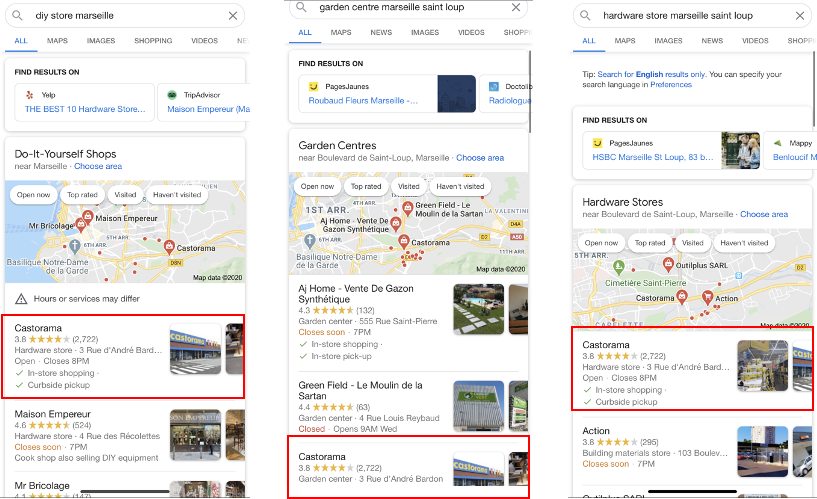Here is a detailed and cleaned-up caption for the image described:

---

The image comprises three side-by-side screenshots of Google search results for various queries related to retailers in Marseille. 

1. The left screenshot displays the results for "DIY store Marseille." It shows multiple sections like Maps, Images, Shopping, and Videos, with the "All" tab highlighted in blue. The first suggestion is "Find results on Yelp," followed by "Do-it-yourself shops" featuring Google Maps with selected options. The search results include Castorama, Maison Empereur, and Mr. Bricolage, with Castorama notably highlighted by a red selection square.

2. The center screenshot is for the search query "Garden Center Marseille St. Loup." Similar to the first, it includes a map and a "Find results on other sites" section. The results once again feature Castorama, which is highlighted.

3. The right screenshot pertains to "Hardware store Marseille St. Loup." Consistent with the other searches, it has sections like Maps and fine results. The options in this search include Castorama and Action, with Castorama prominently selected once more.

Each screenshot consistently highlights Castorama across different search queries for clarity and emphasis.